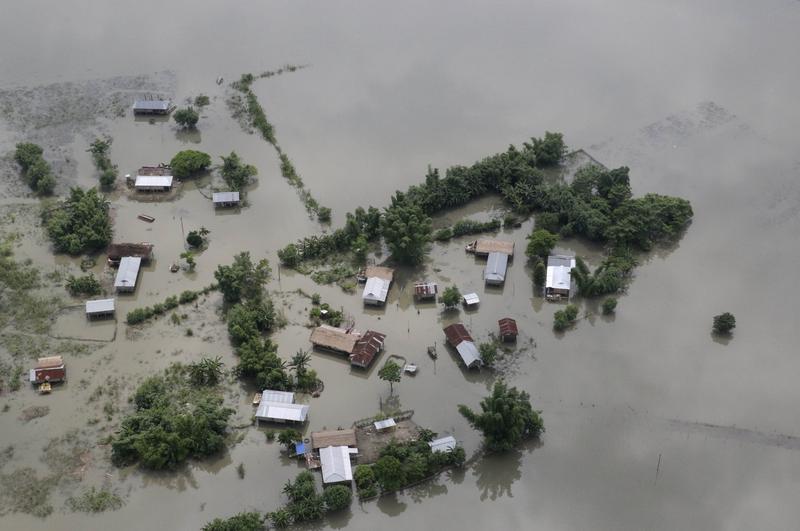The image captures a devastating scene of a flooded area, seemingly taken from a low-flying plane or high-flying drone at around 1,000 feet. The landscape is dominated almost entirely by water, engulfing numerous houses, barns, mobile homes, and sheds. Only the top floors and roofs of these structures are visible, showcasing a variety of materials—metal, red, and brown roofs. The layout of these buildings appears random and unorganized, scattered haphazardly across the scene without any discernible grid pattern. 

Surrounding these submerged structures are clusters of dark green trees, sprouting from what was once solid ground. There's an overwhelming sense of isolation as no people are visible, only buildings marooned in the murky, grayish-blue floodwaters. In the upper left and lower left corners, there are small patches of exposed dirt possibly indicating receding floodwaters, but these are minimal compared to the extensive flooding in the rest of the image. Cars can be seen stranded in the water, adding to the chaotic mix of diverse structures, many appearing old and in poor condition. This aerial view grimly highlights the extensive damage and the randomness with which nature has scattered its wrath.